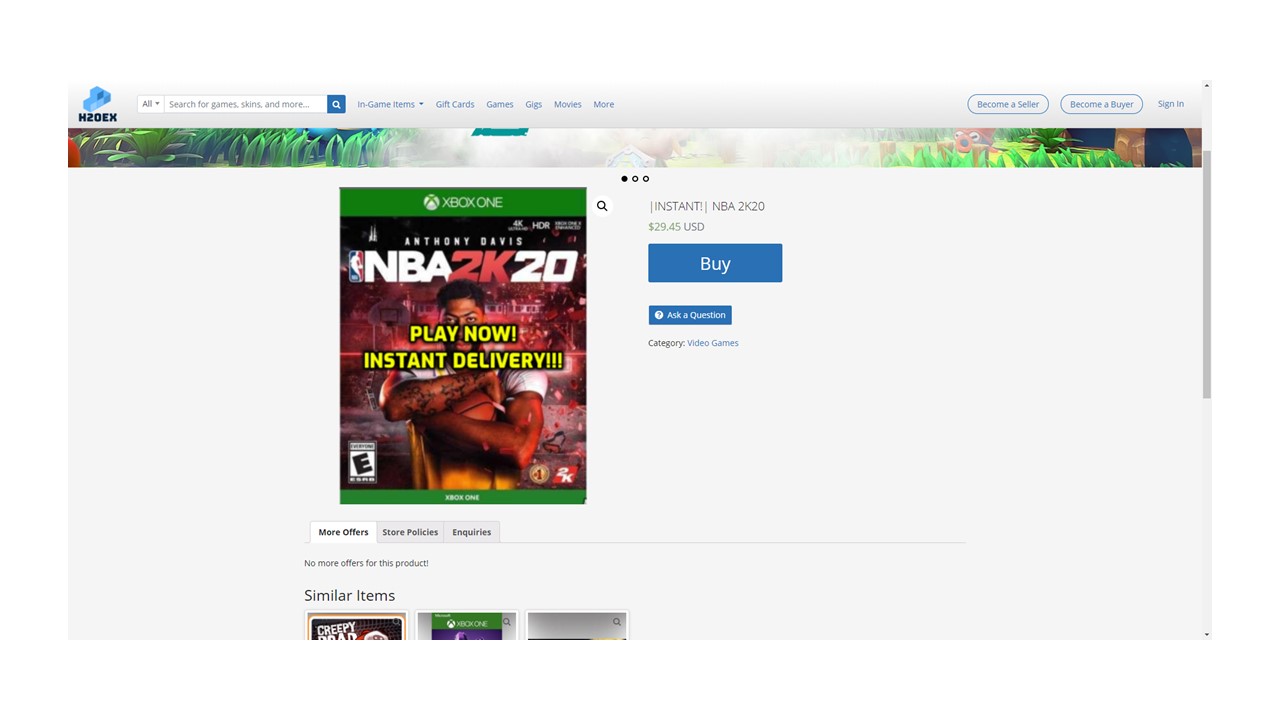The image depicts a scene of purchasing an online game on a laptop or personal computer, using a platform that closely resembles Steam. Displayed prominently on the screen is the game NBA 2K20, specifically the Xbox One version. Toward the right side of the screen, you can see the price listed as $29.45 USD along with a buy icon.

Below the game information, there are three distinct sections labeled: "More Offers," "Store Policies," and "Inquiries." Further beneath these sections, the platform provides a selection of similar items for the user to consider.

At the very top of the screen, there is a colorful banner reminiscent of a cartoon game, featuring a grassy landscape. The top left corner houses a search bar and the platform’s name, H2OEX. Moving your gaze towards the top right corner, you will find buttons for signing in and options to register as either a seller or a buyer.